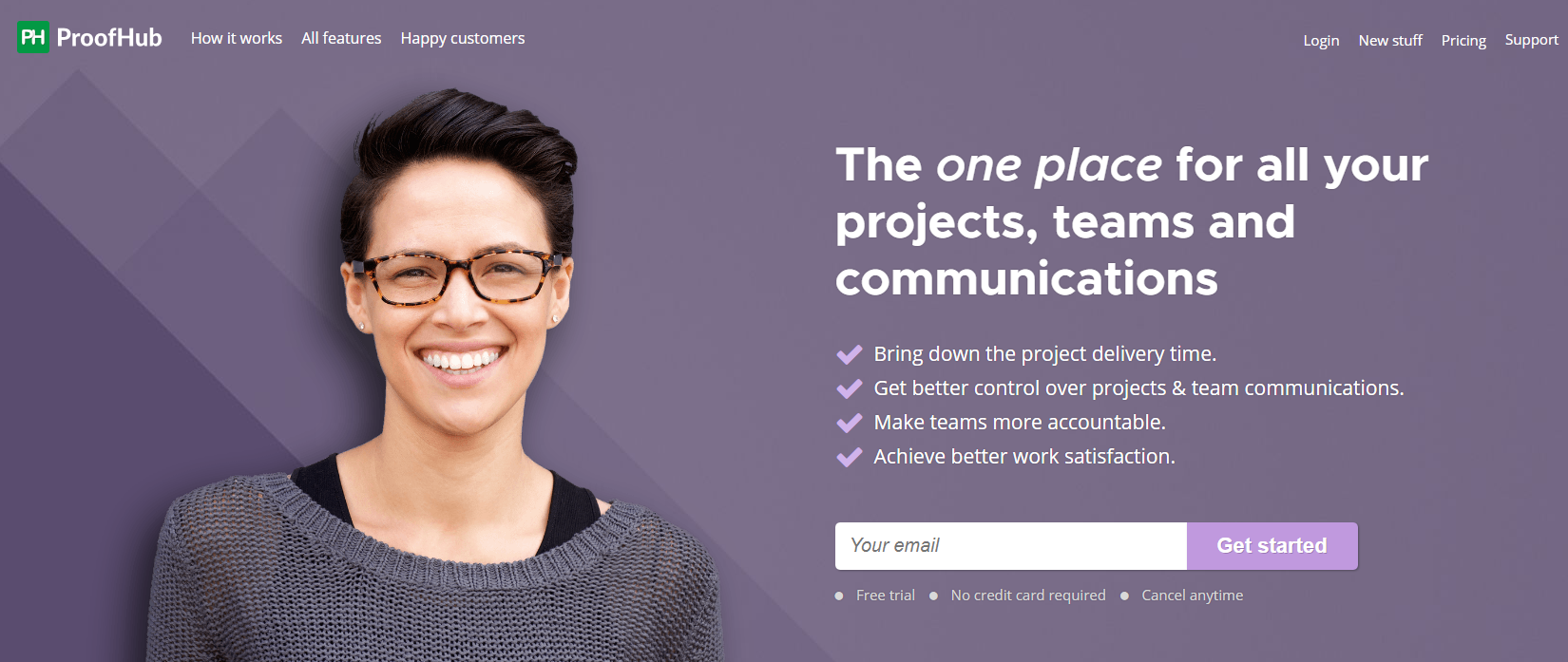This screenshot features the main webpage of Proofhub, a project management website. The page is designed with a light to medium purple background, consistent throughout, revealing the brand's color scheme. The visual center of the page showcases a smiling woman, visible from the shoulders up, gazing directly at the camera. Overlaid on the purple background, white text stands out, incorporating varying shades of purple to enhance the tonal depth.

In the top left corner of the page, a green box presents the white initials "PH," signifying the Proofhub logo. Adjacent to this, the brand name "Proofhub" is displayed, with both 'P' and 'H' capitalized and merged into a single word. The header navigation includes options labeled "How it Works," "All Features," and "Happy Customers" on the left, while the right side features "Login," "New Stuff," "Pricing," and "Support."

A prominent headline in large white letters declares, "The one place for all your projects, teams, and communications." Below this, an additional section lists four benefit-driven statements accompanied by checkmarks in a contrasting purple shade: 
1. Bring down the project delivery time,
2. Get better control over projects and team communications,
3. Make teams more accountable, 
4. Achieve better work satisfaction.

Towards the bottom of this section, a text box invites users to enter their email to "Get Started," encouraging them to initiate their Proofhub journey.